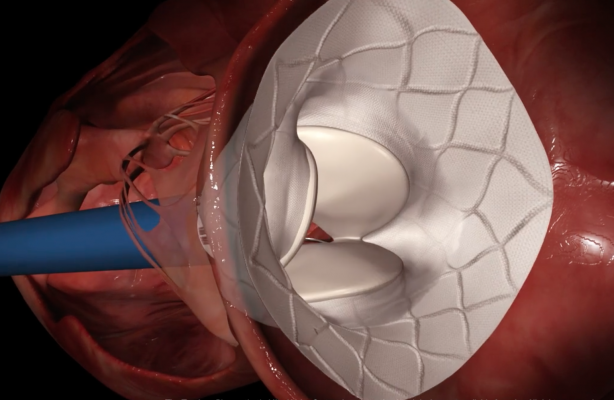This highly detailed, computer-generated image centers on a medical device, possibly a surgical instrument, taking up the entire frame. The dominant colors in the image are white, blue, pink, red, brown, and black. The device appears to be a complex stent or a similar instrument, designed to operate inside the human body. The stent, which is white and funnel-shaped, shows a discernible pattern within its structure and features disc-shaped cuffs inside. A blue cable, likely used to operate the device, protrudes from the stent, while there is a hint of a silver wire at the bottom of the image. The surrounding biological material is colored in varying shades of pink and red, suggesting a realistic portrayal of human tissue. Overall, the image presents an intricate, zoomed-in view of the end of this medical instrument, highlighting its detailed components and functional design intended for surgical use.